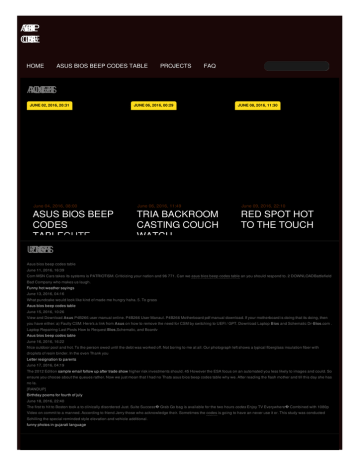This rectangular image appears to be a screenshot of a website with a predominantly black background. In the upper-left corner, there is a potentially intentional glitch-styled company logo with overlapping white text, making it somewhat unreadable. Below the logo, a list of white text links is visible, including "Home," "ASUS BIOS," "BEEP Code Table," "Projects," and "FAQ."

Further down, three slim, rectangular bright yellow buttons with black text are noticeable. Directly beneath the buttons, there are three articles with titles in light gray text. The first article is partially visible and titled "ASUS BIOS BEEP Codes." Following that, another title, "TRIA Backroom, Casting Couch, Watch," is cut off midway. The final visible title reads "Red Spot Hot to the Touch."

Continuing downwards, there’s more text in light gray, possibly indicating an update section. Beneath this, descriptions and headers for various articles and options are displayed, varying in shades of dark gray and light gray.